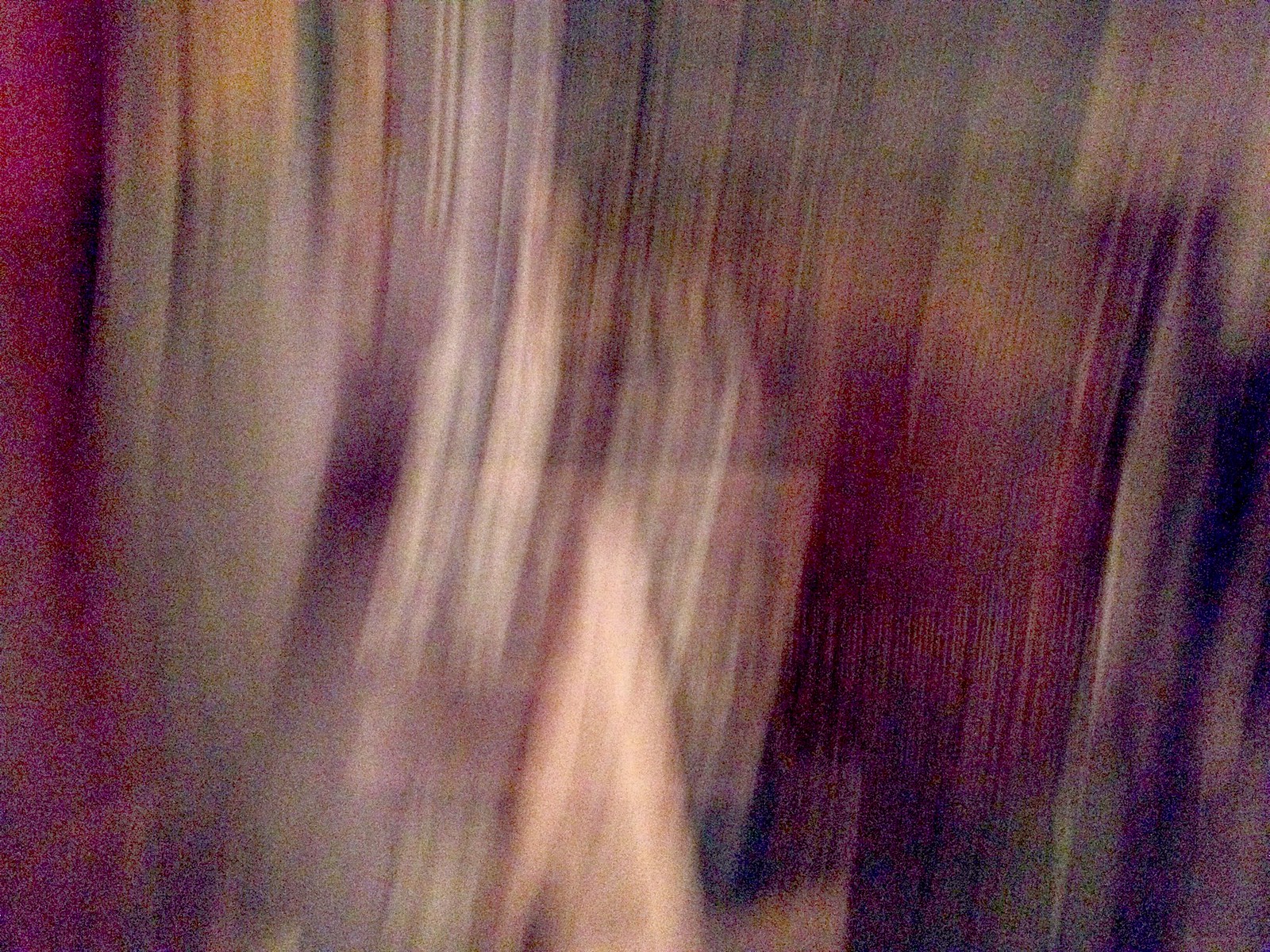The image depicts a highly blurred scene with noticeable horizontal and vertical streaks of various colors, including reddish-brown, tan, green, purple, almost red, black, and goldish-orange. The overall composition gives an abstract and dynamic feel, possibly suggesting rapid movement during the capture. The colors flip-flop between reddish-brown and tan with green mixed intermittently, creating a layered effect. In the central region, approximately 40% from the left and midway downwards, there is a discernible structure resembling a series of gray boxes, extending vertically and nearly half the height of the image. This area may also include a triangular lighter gold or yellowish shape near the bottom center. The blurred nature makes it difficult to determine whether the scene is a real-life setting, such as the inside of a building with tall wood paneling in varied tones, or a digitally created abstract illustration.